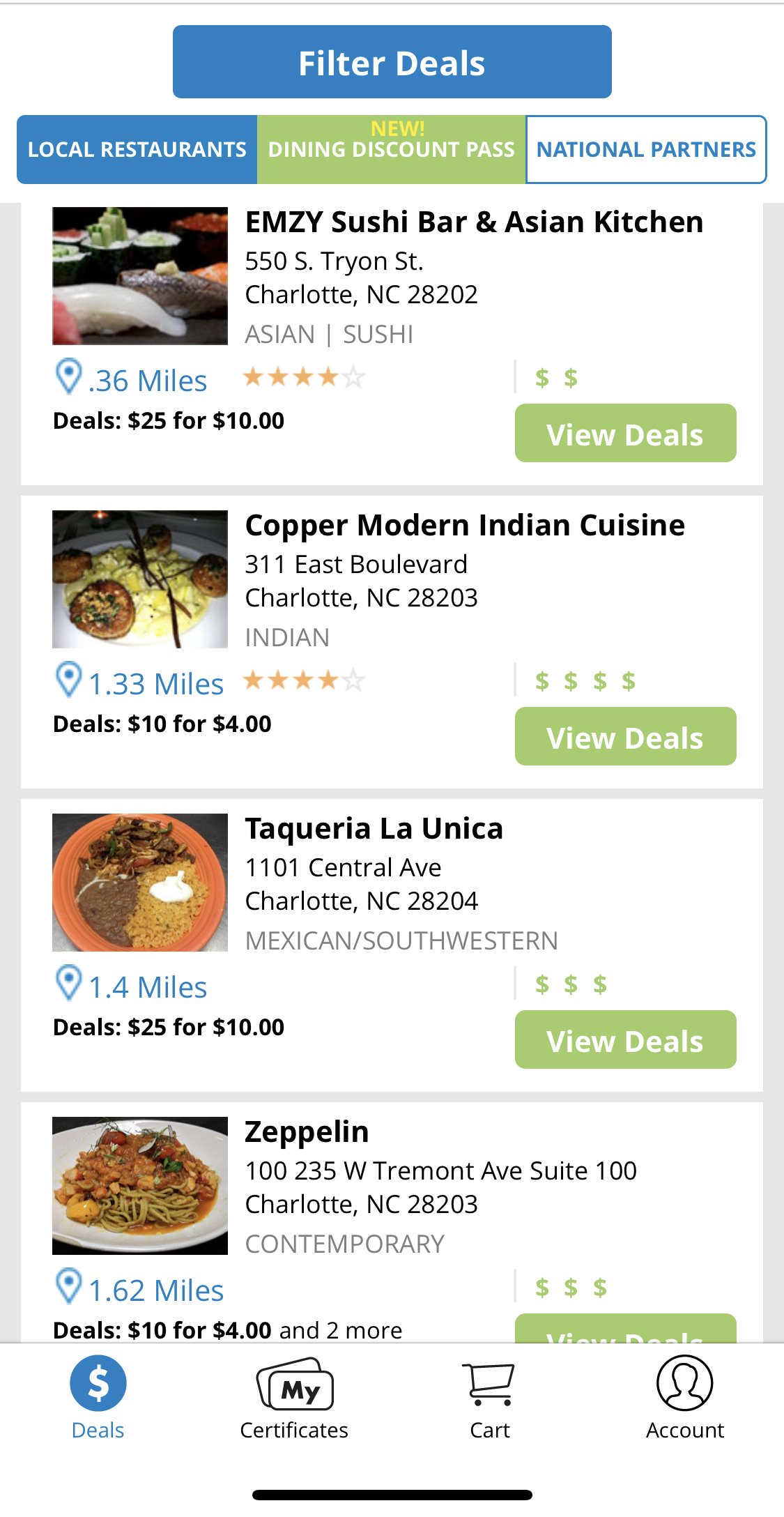This is a screenshot of a dining website showcasing various restaurant deals and offers. At the top of the page, there is a blue navigation bar labeled "Filter Deals". Directly beneath this is another blue tab that says "Local Restaurants". Following this tab, there is a section for "New Discount Passes," and underneath that, a section for "National Partners". 

In the main content area, four restaurant listings are displayed, presumably based on proximity, although no specific location is listed. The restaurants include:
1. MZ Sushi Bar and Asian Kitchen, located 0.36 miles away.
2. Copper Modern Indian Cuisine, located 1.33 miles away.
3. Tequila La Unica, located 1.4 miles away.
4. Zeppelin, located 1.62 miles away.